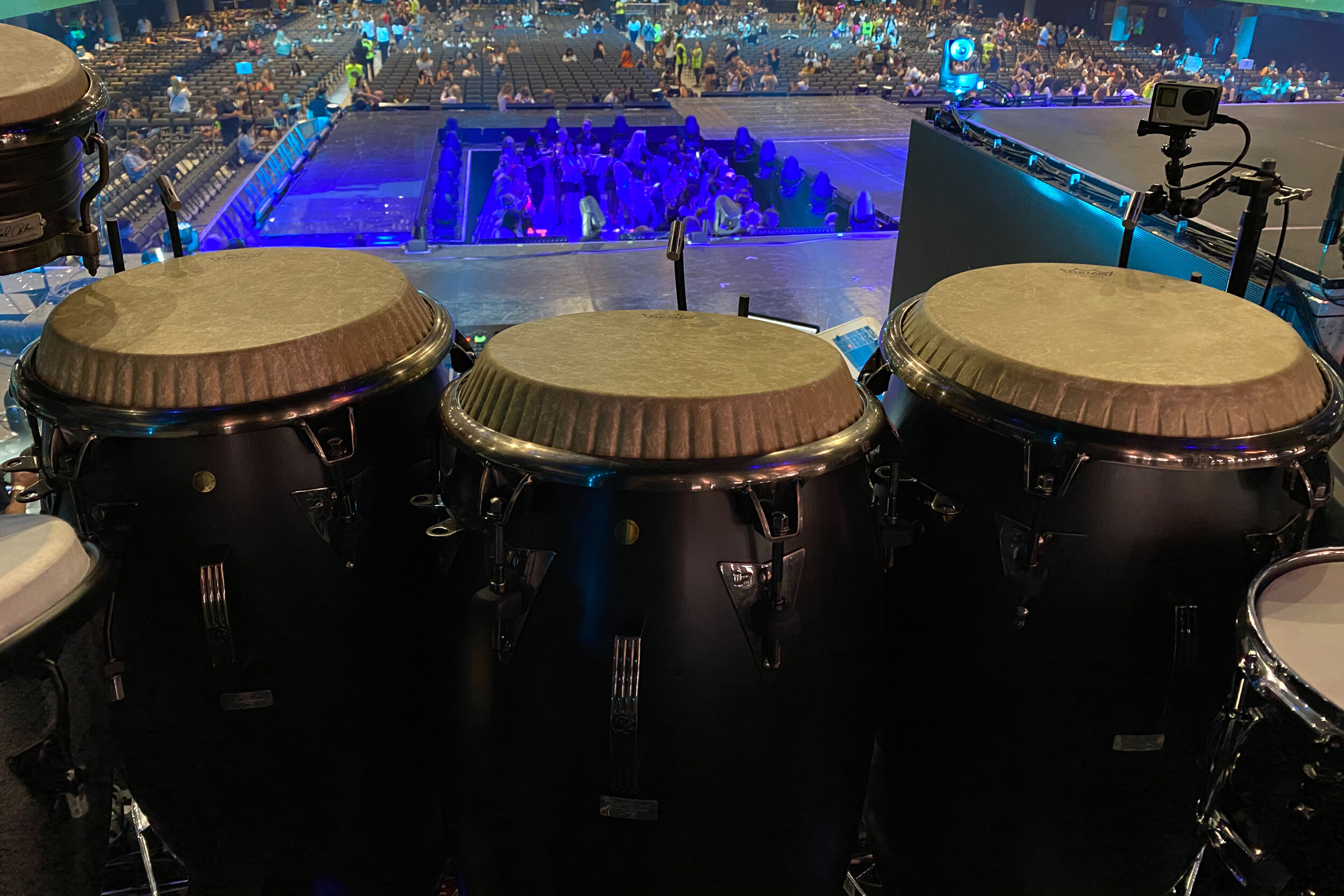The image depicts the point of view of someone positioned behind a set of six varied drums, primarily featuring bongo drums, with tan tops and black and metal bases. The foreground showcases a close-up of these drums, arranged from left to right, and a smaller snare drum on the lower right. To the lower left is part of a chair, emphasizing the stage setup. Adjacent to the drums, a video camera is set up in the upper right-hand corner, suggesting the preparation for an event. In the background, a large stage dominates the scene, bordered by chairs that encircle the stage area. The chairs are only partially occupied, with a sparse but eager audience visible, hinting at an upcoming concert. The image includes a variety of colors—tan, black, gray, blue, green, and hints of orange—completing the scene of anticipation and readiness for a performance.